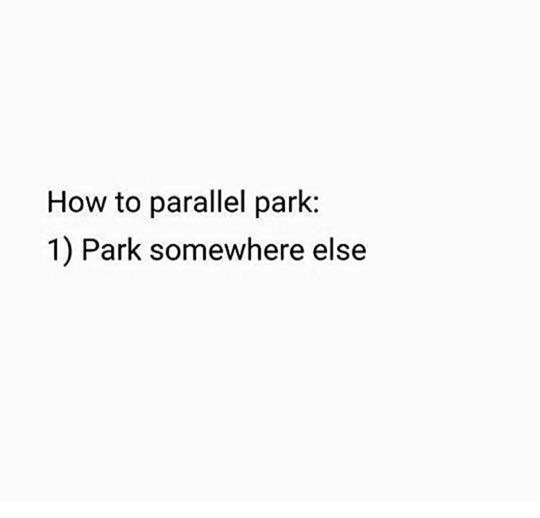The image is a straightforward, text-based meme featuring concise, black printed instructions on a plain white background. At the top, it reads "How to Parallel Park" in capitalized black letters, followed by a colon. Below this title, it lists a single step: "1. Park Somewhere Else," with both "Park" and the first word of the title, "How," capitalized. The overall design is minimalist, with the text centered and surrounded by ample blank space, highlighting the humorous directive.